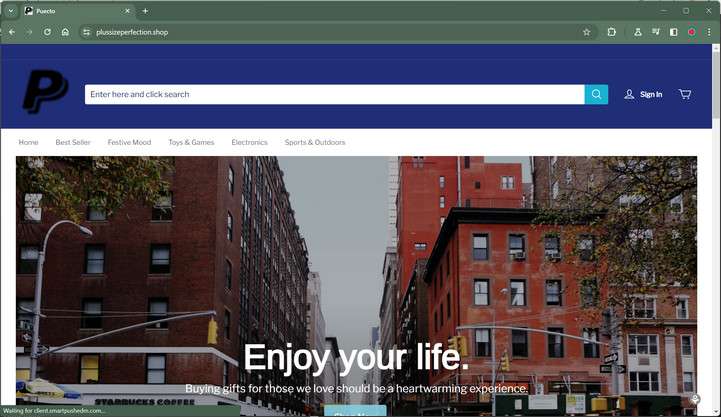The image is a screenshot of the homepage of the website "plussizeperfection.shop." At the top of the page, there's a gray navigation bar followed by a large, navy blue strip extending horizontally across the screen. On the left side of the strip, there is a prominent black letter "P" which serves as the logo for the site. Adjacent to the logo, a lengthy search bar with the placeholder text "Enter here and click search" is flanked by a blue search button. To the right of the search bar, options for "Sign In" and a shopping cart icon are visible.

Beneath this, the rest of the page features a white background. At the top of this section, there is a menu bar with the following categories: Home, Bestseller, Festive Mood, Toys and Games, Electronics, and Sports and Outdoors.

A large banner image dominates the main section of the page just below the menu bar. On the left side of the banner, there is a view of a brownish brick building, while the right side showcases a collection of red buildings of various sizes. The scene includes city elements such as traffic lights. Overlaid on this image is white text that reads "Enjoy your life." Below this in smaller text, it states, "Buying gifts for those we love should be a heartwarming experience."